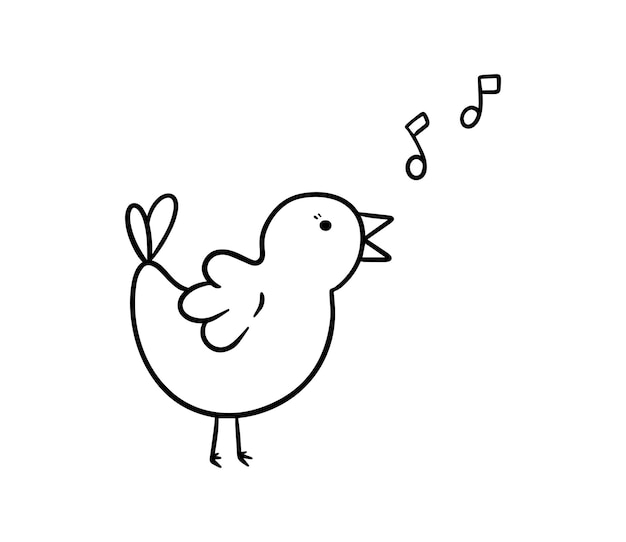The image features a simplistic, cartoon-like drawing of a small chick, rendered in black and white line art, with no color or additional background elements. The chick is depicted in a profile view with one tiny black dot for its eye and two short lines for eyelashes. Its open beak is drawn as two spread-apart triangles, and from its beak rise two musical notes, suggesting that the chick is singing. The chick's wing, resembling a three-fingered hand or a cartoon glove, is spread out. It has a tail composed of two teardrop-shaped feathers. The little chick stands on two extremely thin legs with feet that each have three tiny toes. Overall, the image is a simple, hand-drawn or digitally-stylized piece showing a cheerful, singing cartoon chick against a plain white background.